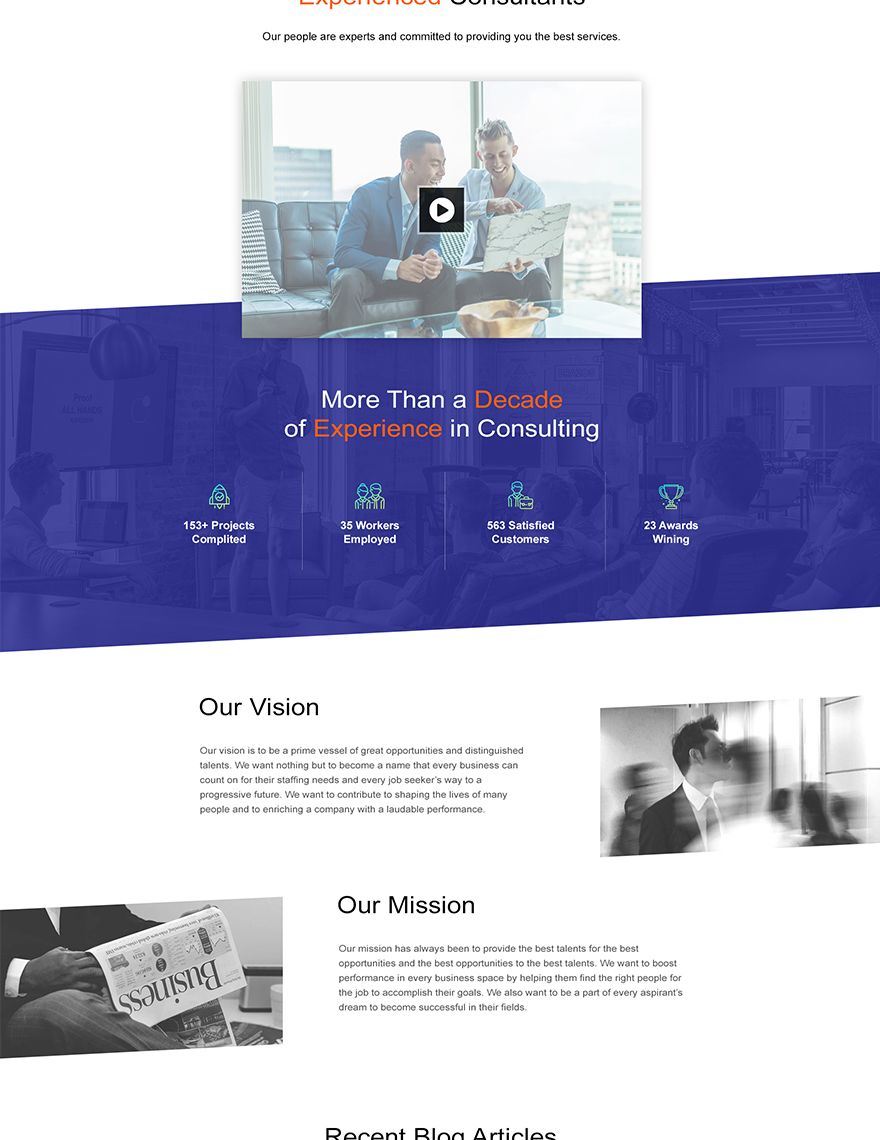The image appears to be of a business consulting firm's webpage. At the top, the text prominently declares, "Our people are experts and committed to providing you the best services." Directly below this headline is a video with a play button in its center. The still frame from the video features a photograph of two men sitting on a couch, both intently focused on a laptop in front of them. Behind the men, a cityscape can be seen, indicating that they are likely inside an office building with large windows.

Further down, there is a blue box showcasing some key statistics: "More than a decade of experience in consulting. 153+ projects completed. 35 workers employed. 563 satisfied customers. 23 awards won." This section emphasizes the firm's extensive experience and achievements.

The next section is titled "Our Vision," accompanied by a detailed description: "Our vision is to be a prime vessel of great opportunities and distinguished talents. We want nothing but to become a name that every business can count on for their staffing needs and every job seeker's way to a progressive future. We want to contribute to shaping the lives of many people into enriching a company with a laudable performance."

To the right of "Our Vision," there is a somewhat blurred side-view photograph of a man. Beneath this image is the heading "Our Mission," with corresponding text detailing the firm's mission. To the left, another photograph centers on a newspaper business page with the caption "Recent Blog Articles."

Overall, this webpage effectively showcases the consulting firm's expertise, experience, and commitment to its clients and stakeholders.